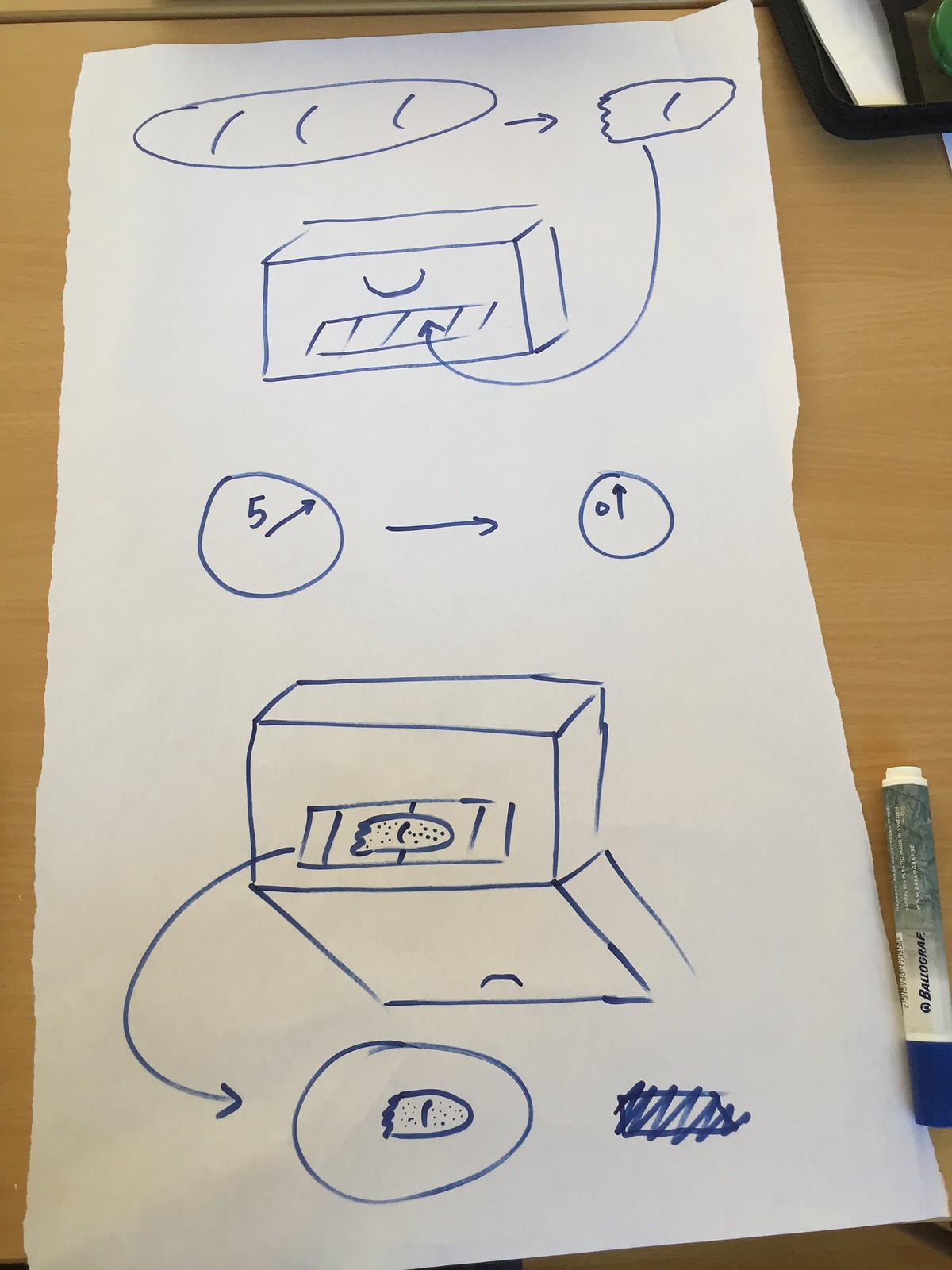The photograph is a vertically oriented, full-color image showcasing a white piece of paper placed on a wooden table. The paper appears to be torn along its left and right edges and is positioned with a slight diagonal slant. On this paper, there is a hand-drawn diagram that seems to outline a process or set of instructions.

In the upper section of the paper, there is a simple sketch featuring a loaf of bread on the left, connected by an arrow to a half-broken loaf of bread. This arrow points into a rectangular shape, resembling an oven, and likely represents the first step of the process.

Beneath this, there is a circle labeled with the number "5" and an arrow. In the center of this area, another arrow points to the right towards an adjacent circle labeled with "0", possibly indicating the duration the bread should be placed in the oven—perhaps five minutes or five hours.

Lower down, the diagram depicts another rectangular shape, again symbolizing an oven, but this time with the door open. A curved arrow indicates the bread, now dotted to show it's baked, being taken out. Adjacent to this oven illustration is a circular shape representing a plate, on which the half piece of bread is now placed.

In the bottom right corner of the photograph, a marker lies on the wooden table, suggesting the diagram was recently sketched.